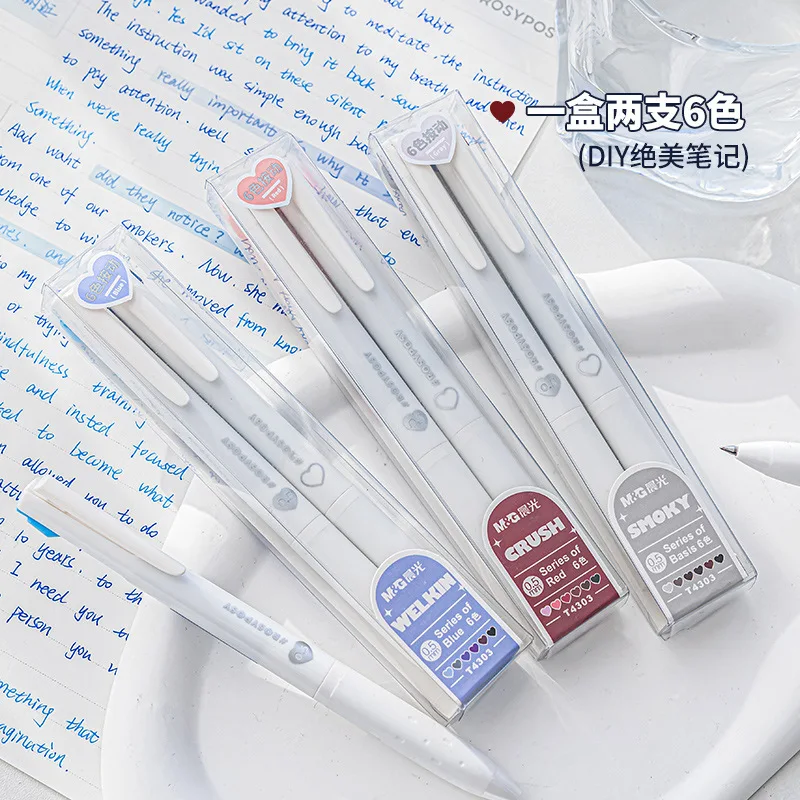The image is a detailed photograph, likely an advertisement for ink pen products. At the top right corner, there are distinctive Asian characters in white next to a small, solid red heart. Below this, in black letters, is the text "D.I.Y." followed by more Asian characters. The central focus of the image is on three long, plastic containers, each containing a black rod, which appear to be different colored pen inserts. The containers vary in color at the bottom: the left one is light blue labeled "Welchem," the middle one is red labeled "Crush," and the right one is grey labeled "Smokey." To the left of these containers, there is a pen pointing downwards, and another pen's point is visible coming in from the right center. Behind these containers, a white piece of paper with indiscernible blue text is visible, adding to the impression that these products are oriented towards writing or artistic functions.